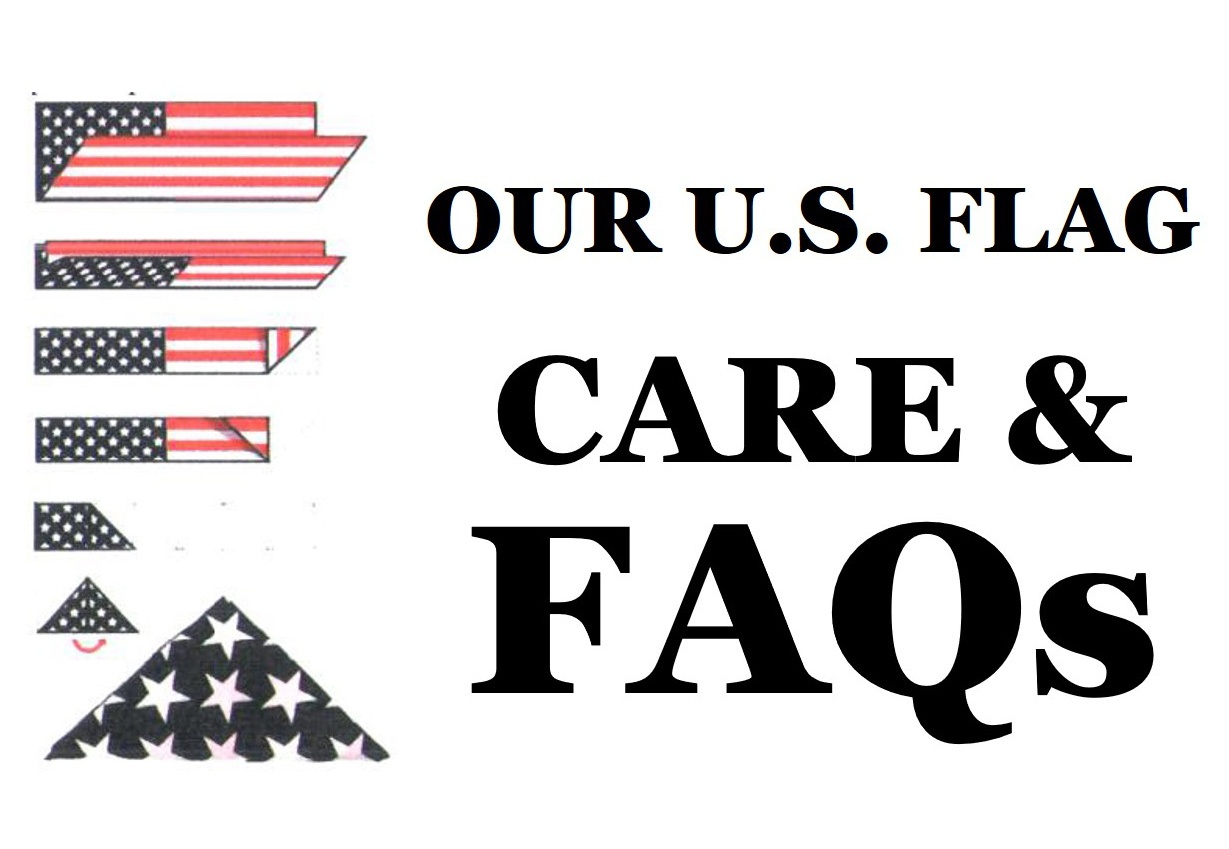The image features a step-by-step visual guide on how to properly fold an American flag, set against a predominantly white background. On the left side, a series of pictures illustrate the folding process: starting with an American flag almost folded in half at the top, followed by successive images showing further folds until it forms a perfect triangle with only the blue field of white stars visible. To the right of these instructional images is bold black text that reads, "Our U.S. Flag. Care and FAQs." The text implies that the image might be part of a larger resource dedicated to flag care and frequently asked questions about proper flag handling.